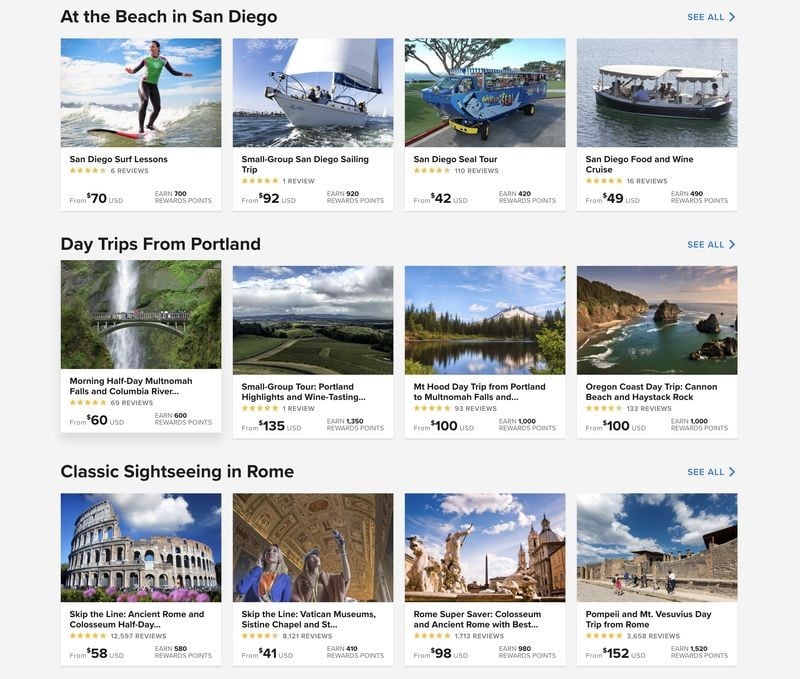The image is a screenshot from a desktop website showcasing a diverse collection of activity recommendations spanning various global locations, including San Diego, Portland, and Rome. At the top of the image, San Diego features several beach-related activities such as surf lessons, a sailing trip, a seal tour, and a food and wine cruise. Each activity is accompanied by details such as the cost in U.S. dollars, the number of reviews, and the reward points that can be earned.

Beneath the San Diego activities, there are multiple day trips from Portland, including a morning half-day trip to Multnomah Falls and Columbia River Gorge, a group tour highlighting wine tasting, a day trip to Mount Hood with a stop at Multnomah Falls, and an Oregon Coast day trip to Cannon Beach and Haystack Rock.

Finally, the image presents sightseeing options in Rome, further contributing to the variety of activities available across different locations. The screenshot effectively illustrates the range of travel experiences from beach outings in San Diego to scenic adventures in Portland and cultural explorations in Rome.